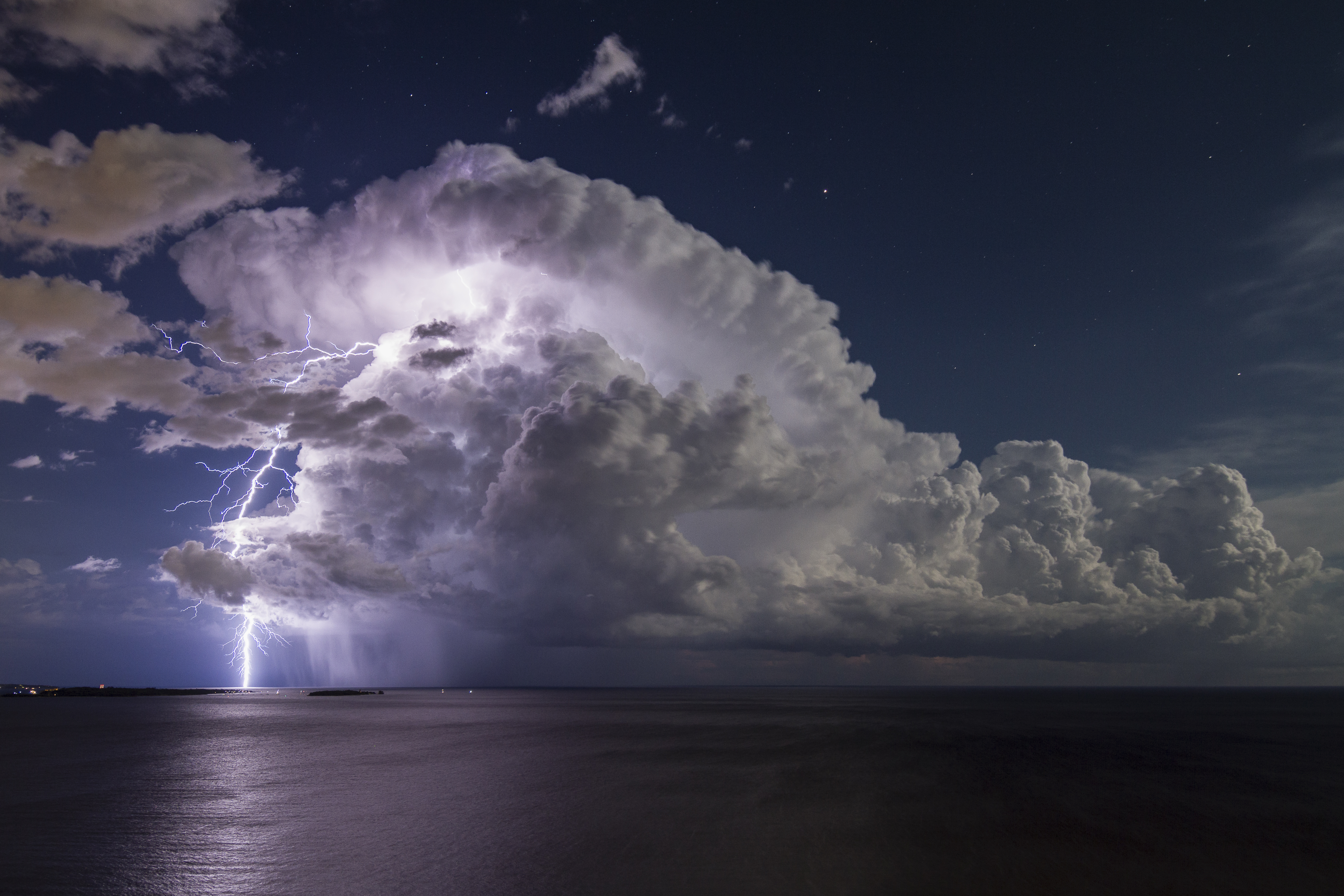This is a dramatic nighttime photograph capturing a spectacular lightning storm over the ocean. The sky is dominated by a massive, thick cloud formation, predominantly gray with sections illuminated to a brilliant white by the lightning bolts. The largest and most striking cloud is positioned slightly to the left of center and extends across the sky. The lightning electrifies this main cloud and highlights just how detailed and thick it is, with bolts striking both downward into the water and upward into the misty atmosphere above.

The ocean beneath looks almost black, with its smooth, reflective surface subtly illuminated by the bright flashes of lightning. The distant scene creates a sense of vastness, with the storm and its dramatic elements appearing far off but intensely visible. Smaller clouds flank the main formation, with some billowy clouds to the right. The combination of the dark sky, the varied textures of the clouds, and the vivid lightning strikes make this one of the most incredible and visually stunning storm photographs ever seen.